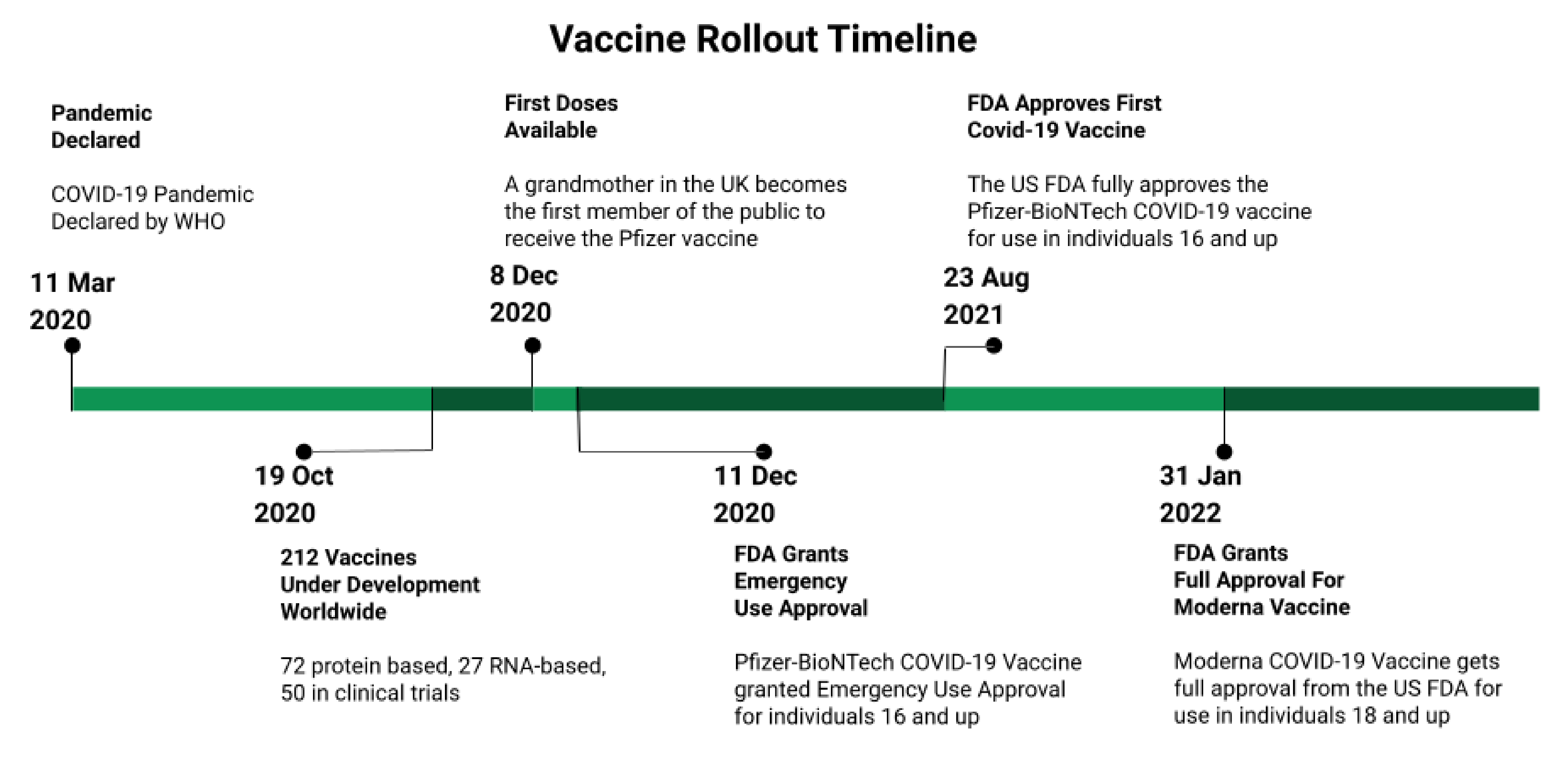The image is a detailed timeline of the COVID-19 vaccine rollout, starting from the pandemic declaration to the full approval of vaccines. At the top center, the title "Vaccine Rollout Timeline" is prominently displayed in black text against a white background. The timeline begins on the left with the date 11 March 2020, when the COVID-19 pandemic was declared by the World Health Organization (WHO). A green horizontal bar runs through the middle of the image with various milestone dates and corresponding descriptions marked along it.

On 19 October 2020, 212 vaccines were under development worldwide, consisting of 72 protein-based and 27 RNA-based vaccines, with 15 of these in clinical trials. 

Moving forward, on 8 December 2020, the first doses of the Pfizer vaccine became available, and a grandmother in the UK was the first member of the public to receive it. 

Shortly after, on 11 December 2020, the FDA granted emergency use approval for the Pfizer-BioNTech COVID-19 vaccine for individuals 16 and older. 

Continuing along the timeline, on 23 August 2021, the FDA fully approved the Pfizer-BioNTech COVID-19 vaccine for use in individuals 16 and older. 

Finally, the timeline concludes with the date 31 January 2022, when the FDA granted full approval for the Moderna COVID-19 vaccine for individuals 18 and older. 

Throughout the timeline, green arrows point to significant dates and provide brief descriptions, making the progression of vaccine development and approval clear and easy to follow.